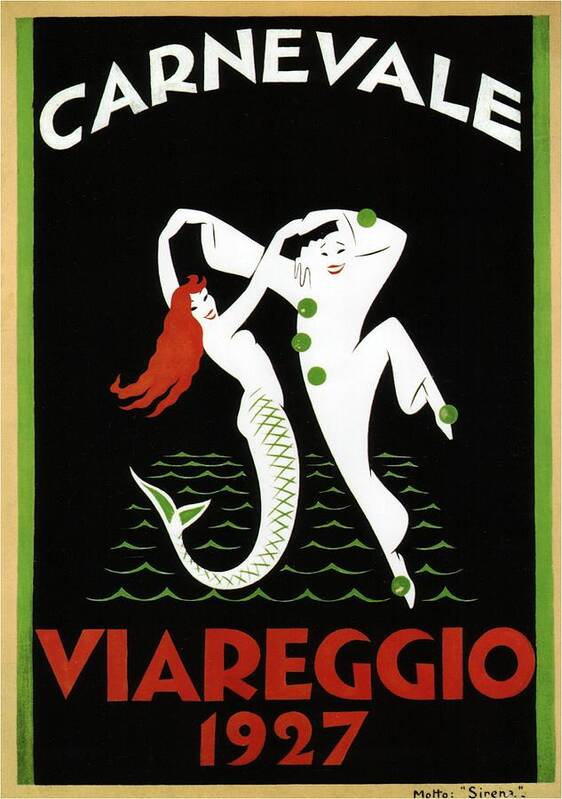This vintage poster, adorned with a matte black background and a beige trim around its edges, advertises an event titled "Carnivale" at the top in bold white letters. At the bottom, in striking red text, it reads "Viriegio 1927". The central image showcases an enchanting scene of a mermaid and a clown dancing atop stylized, wavy green water. The mermaid, with her radiant red hair, smiles joyfully, her tail depicted with delicate green lines and light green stripes. Dancing opposite her is a clown dressed entirely in white, his outfit detailed with green spheres serving as buttons, cufflinks, and decorations on his shoes. The poster's background remains consistently deep black, highlighted by a green border surrounding the central image, contributing to its vibrant and whimsical design.